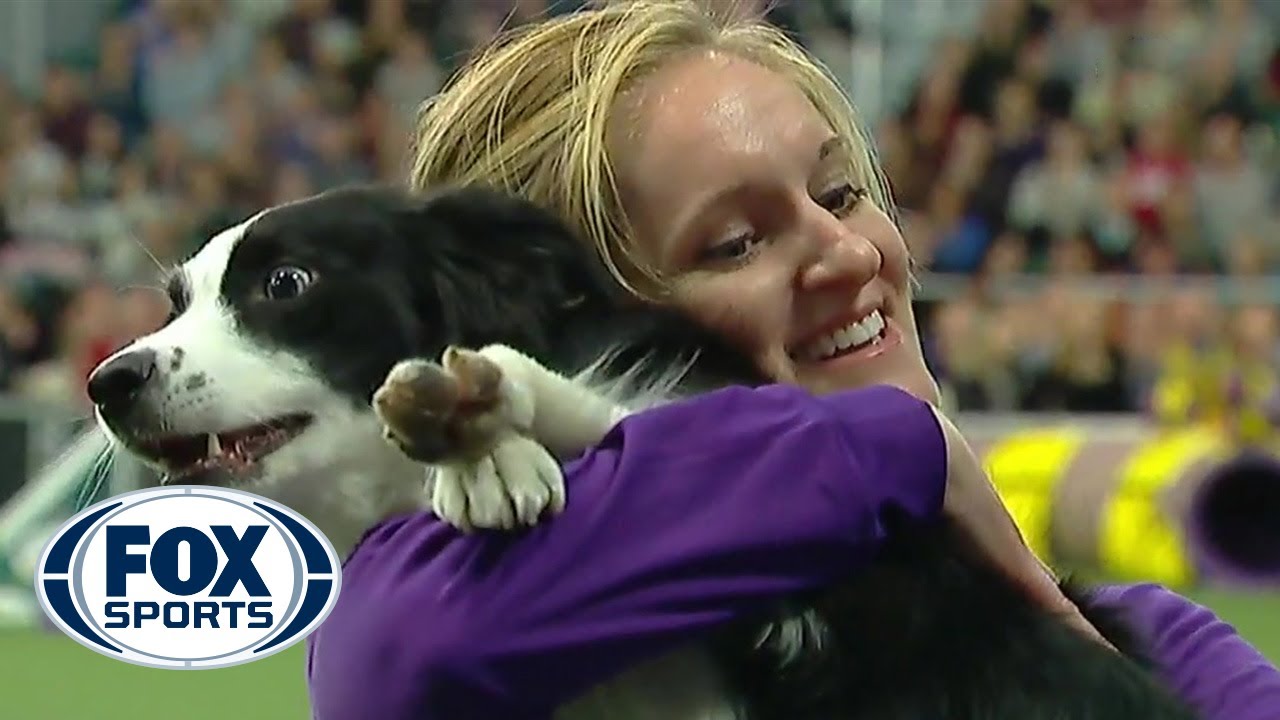This photograph captures a joyful moment of a woman at a dog competition, holding and hugging a Border Collie with a triumphant smile on her face. The woman, who has blonde hair and looks young, is dressed in a purple sweatshirt. The black and white Border Collie, characterized by its mostly black fur with a white face, neck stripe, and white paws, appears to be excited, possibly having just won an event, as suggested by its open mouth and the woman's celebratory demeanor. They are standing on a field, which is evident from the green blurry background, and there are spectators in the stands, also blurred. Notably, the lower left corner of the image features the Fox Sports logo, indicating media coverage. The background also includes some indistinct yellow and purple objects, likely equipment used in the dog competition.